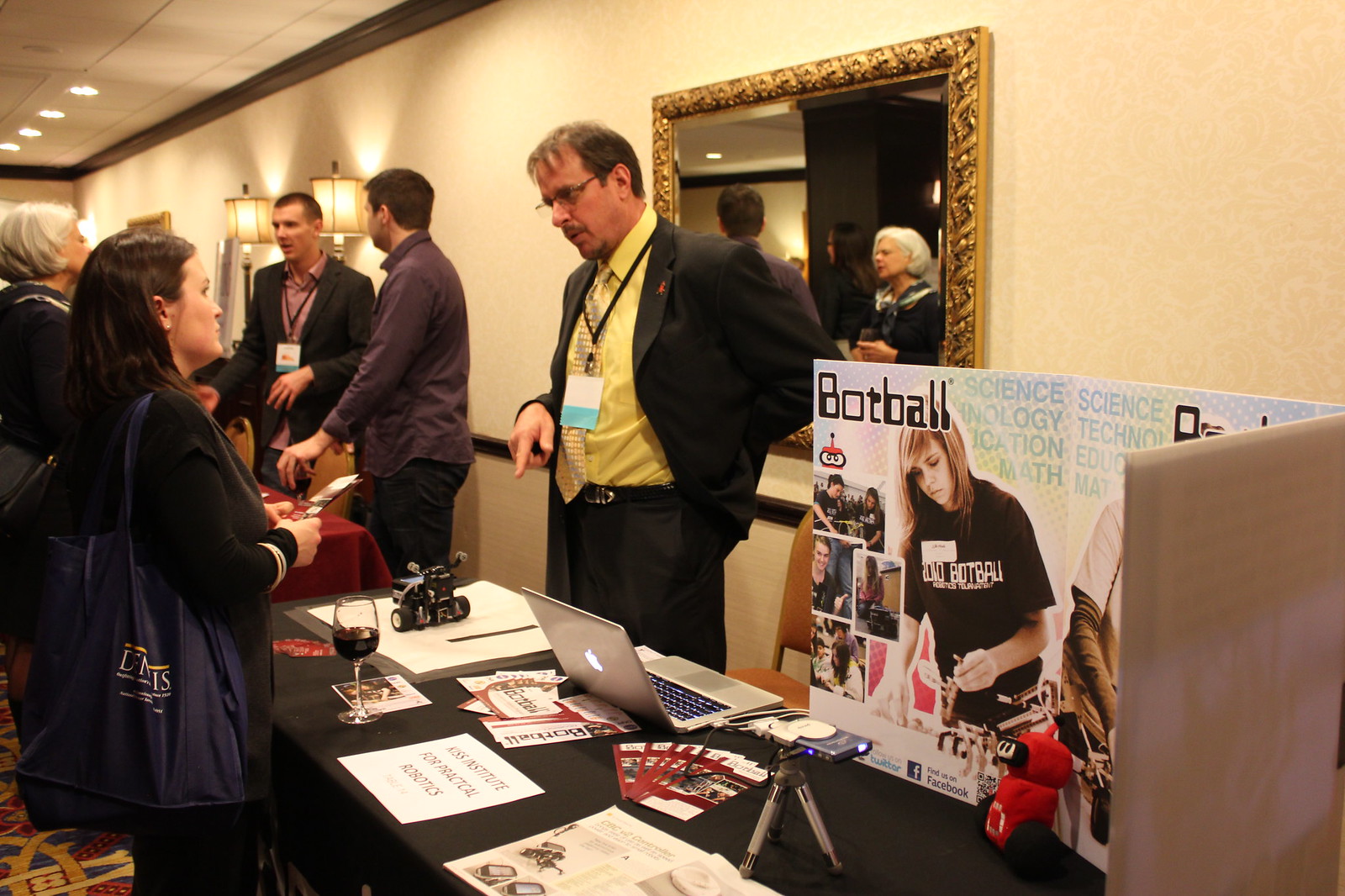This image captures an interior scene of a technology or science-focused exhibition or convention. A man in a black suit, paired with a yellow shirt and a yellow and gray tie with square designs, stands behind a table draped with a black tablecloth. On the table, an open Apple laptop sits next to several flyers and a sign with blue and black lettering that reads "BotBall Science Technology Education Math." A small robotic device with wheels, though not fully detailed, is also present on the table. 

The man appears to be engaging with a woman in a dark coat, holding a pamphlet and a glass of wine, possibly explaining the BotBall concept or answering her questions. The setting includes an ornate, gold-framed mirror on a beige wall, suggesting this might be in a sophisticated space such as a hotel lobby or office environment. Additional tables with exhibitors and attendees are also visible, emphasizing the bustling, interactive atmosphere of the event.